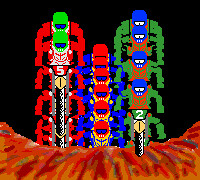This is a small, pixelated digital image, possibly from a video game or a basic paint program, featuring a dirt bike scene. The foreground showcases a brownish-red hill or path curving inwards at the bottom of the screen, illustrated with brush strokes indicating some texture. Three riders on dirt bikes are prominently displayed, seemingly layered and stacked on top of each other in columns. The rider on the left sports red attire with a green helmet, while the middle rider wears blue with a red helmet, and the right rider is in green with a blue helmet. Each column has multiple identical riders, with the left column having around five, the middle possibly up to seven, and the right around four or five. The stark black background makes the colorful riders and their detailed gear, including blue goggles, stand out vividly, creating a unique and layered visual effect.